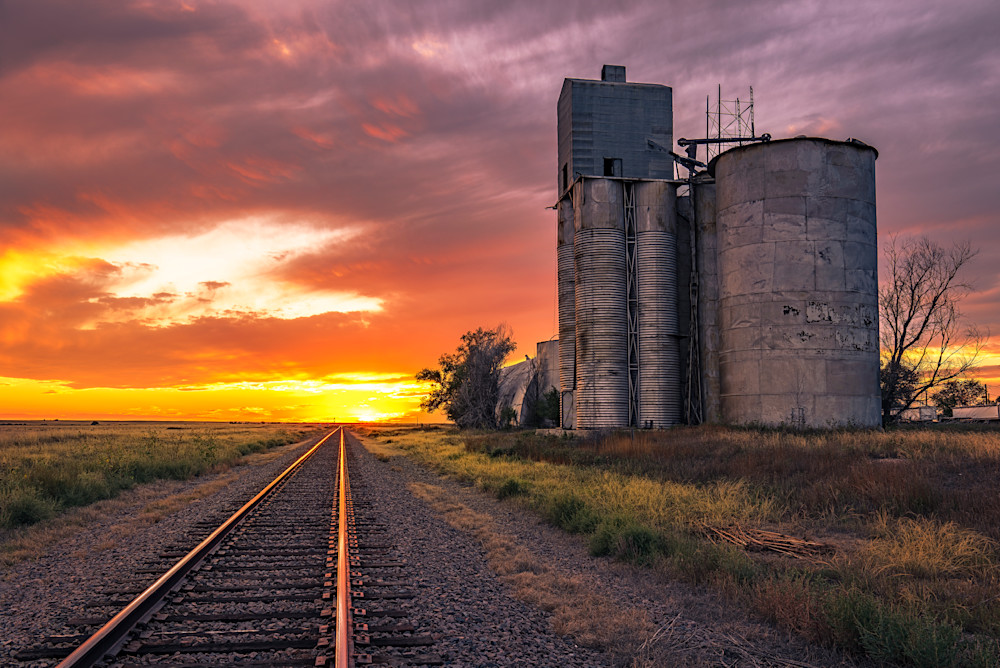The photograph captures a tranquil outdoor scene at sunset, featuring a railroad track that stretches off into the distance towards a golden horizon. The two steel rails, supported by wooden sleepers and set on gray ballast, guide the eye towards the setting sun, which bathes the sky in warm hues of yellow and orange, intermixed with bluish-purple clouds. To the left of the track lies a flat field overgrown with tall, untended grass and bushes, softening the harshness of the industrial elements. On the right side, a silver, weathered metal silo complex stands prominently, composed of three towering cylinders adorned with scaffolding. These structures, made from various metal sheets, appear worn and rustic, contrasting against the colorful, slightly clouded sky behind them. The scene captures a moment of serene beauty and rugged industrial charm, merging nature with man-made constructs.